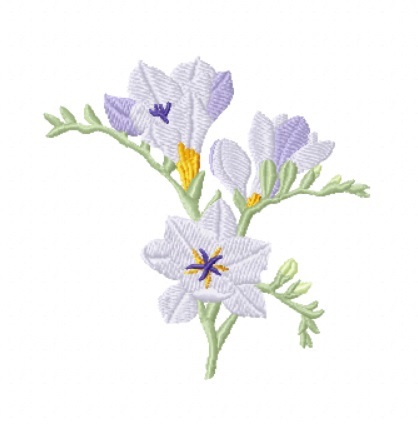The image features an exquisite embroidery of flowers on a completely white background, showcasing detailed and colorful needlework. The primary focus is a series of purple and white flowers with varying shades from light to dark purple, meticulously sewn onto green stems and vines. There are four prominent flower buds, each with intricate detailing, including some with dark purple centers and one with a golden center. Additionally, bright yellow elements are found at the bottom of the flowers and where the pollen would be. The composition of the embroidered vines shows two main branches: one extending from the left to the right and looping back towards the middle, and another smaller one pointing to the right. This needlework beautifully captures the full anatomy of the flowers, from their petals to their stems, showcasing a harmonious blend of light blue, dark blue, medium blue, purple, and yellow hues against a pristine white backdrop.